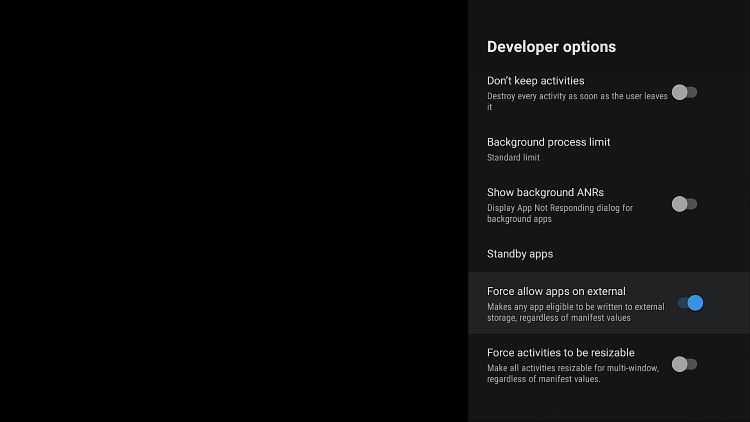Screenshot of Developer Options on a Mobile Device

The image showcases a screenshot of a mobile device's Developer Options settings, displayed against a predominantly black background that transitions to dark gray on the right side. The settings are presented in white text, creating a stark contrast for easy readability.

Highlighted options include:

1. **"Don't keep activities"** - This is designed to destroy every activity as soon as the user leaves it. The associated toggle bar is currently set to 'off'.
  
2. **"Background process limit"** - Set to 'Standard limit' by default.
  
3. **"Show background ANRs"** - ANRs (Application Not Responding) are shown in all uppercase letters, indicating the option to display an ANR dialogue for background apps. This toggle bar is also set to 'off'.
  
4. **"Standby apps"** - Provides management options for standby behaviors of apps.
  
5. **"Force allow apps on external"** - This setting makes any application eligible to be written to external storage regardless of the manifest values set by the app developer. The toggle bar for this option is turned 'on' and is indicated by a blue circle.
  
6. **"Force activities to be resizable"** - Enforces that all activities are resizable for multi-window use, regardless of manifest configurations. This toggle is currently 'off'.

The interface is neatly organized, providing developers with the necessary tools and settings to test and debug applications effectively.